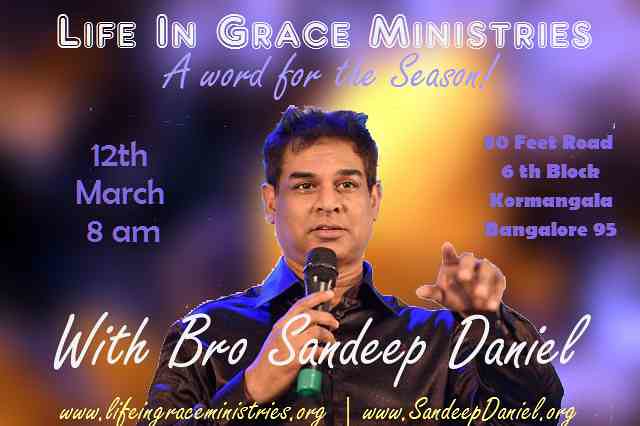The image is an advertisement from Life and Grace Ministries, prominently featuring a middle-aged South Asian man, likely Brother Sandeep Daniel. He has short brown hair and is dressed in a long-sleeved black collared shirt. He is holding a microphone with a green end in one hand and gesturing towards the audience with the other. The background is blurred, emphasizing his figure.

At the top of the image, "Life and Grace Ministries" is written in bold white, bubbly font, while beneath it, "A Word for the Season" is displayed in a cursive purple font. The date and time, "12th March at 8 a.m.", are written in purple on the left side of the image, and the location, "80 or 90 Feet Road, 6th Block, Cormangala, Bangalore 95," is in purple on the right side. At the bottom, in a white cursive font, it reads "With Bro. Sandeep Daniel". Finally, the website "sandeepdaniel.org" is displayed at the very bottom in yellow.